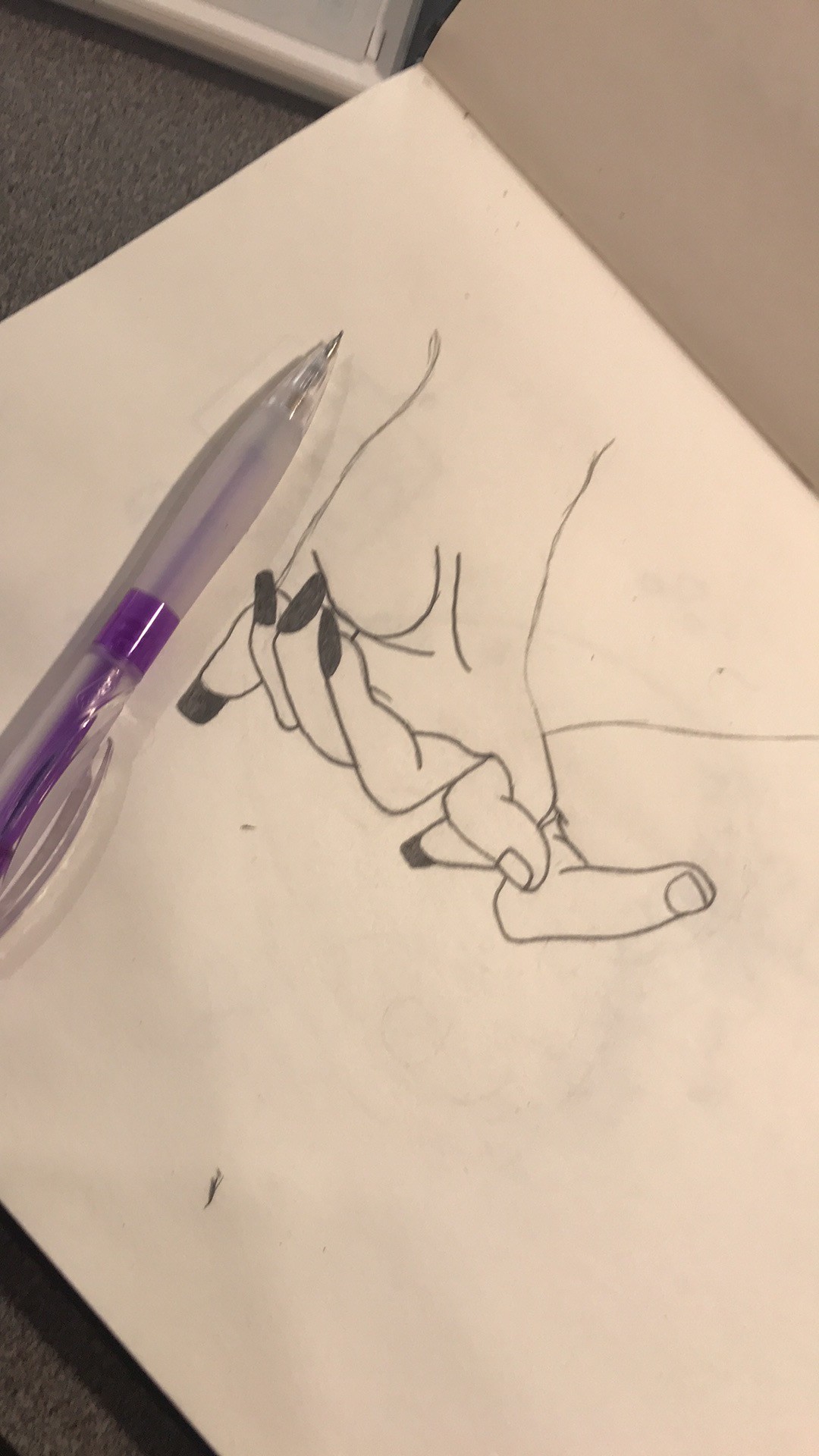On a plain, unlined sheet of paper from a notebook, there is a detailed pen drawing of two hands. The notebook, which lacks a binder, rests on a gray microfiber fabric, possibly part of a sofa or chair. A transparent plastic pen with purple accents and a translucent purple rear portion lies on top of the paper. The drawing depicts one hand with black-painted nails, palm facing up, with the pinky finger extended. A second hand, showcasing only two fingers, grasps onto the extended pinky finger of the first hand.